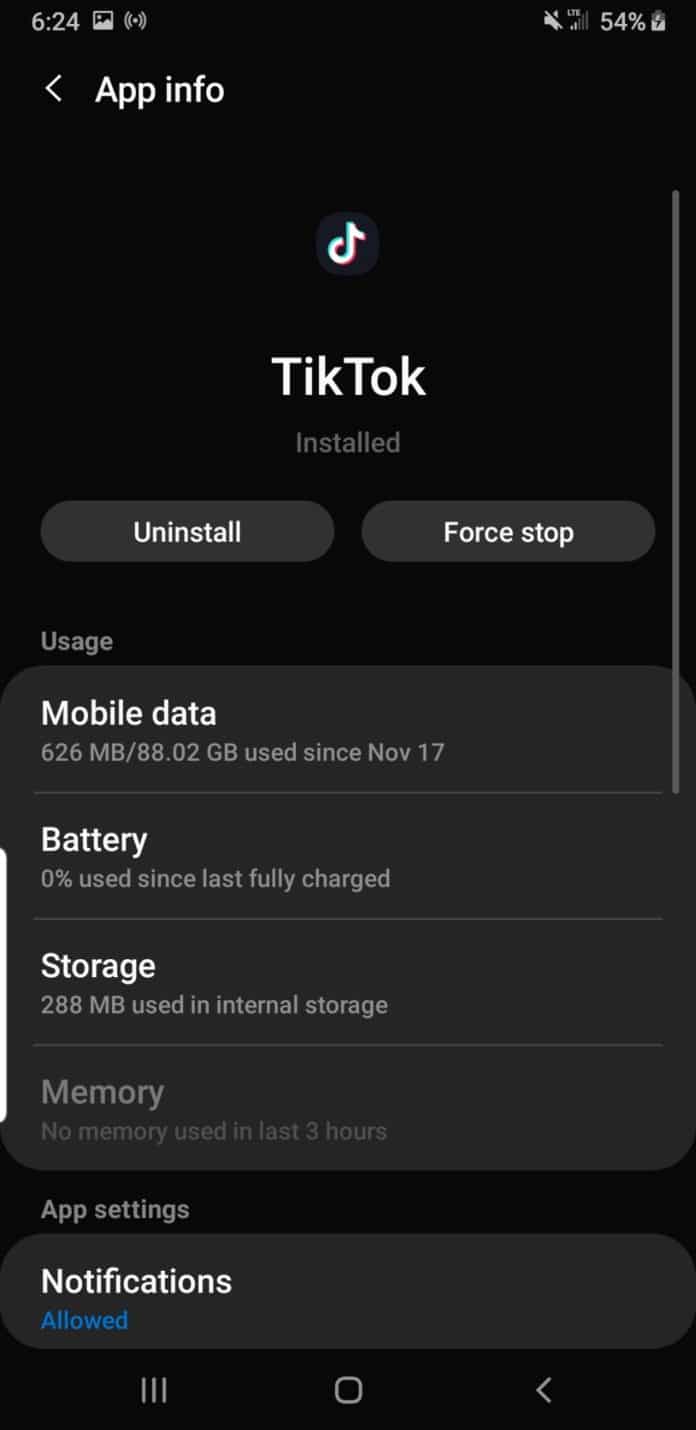The image is a screen capture taken from a mobile device, displaying the 'App Info' page for the TikTok application. The background of the screen is black. In the upper left corner of the screen, the time is shown as 6:24. Directly below the time, the words 'App Info' are written in white. Central to the image is the TikTok icon, accompanied by the text 'TikTok' also in white. 

In the lower left corner, the word 'Allowed' stands out in blue, contrasting with the otherwise white text. Below the TikTok icon, the word 'Installed' is displayed in white text. Underneath 'Installed,' there are two gray buttons. The button on the left is labeled 'Uninstall,' while the button on the right is labeled 'Force Stop.'

Further down the screen, on the left, is the section labeled 'Usage.' Under 'Usage,' larger text indicates 'Mobile Data,' which is followed by smaller text stating, '626 MB / 88.02 GB used since November 17.'